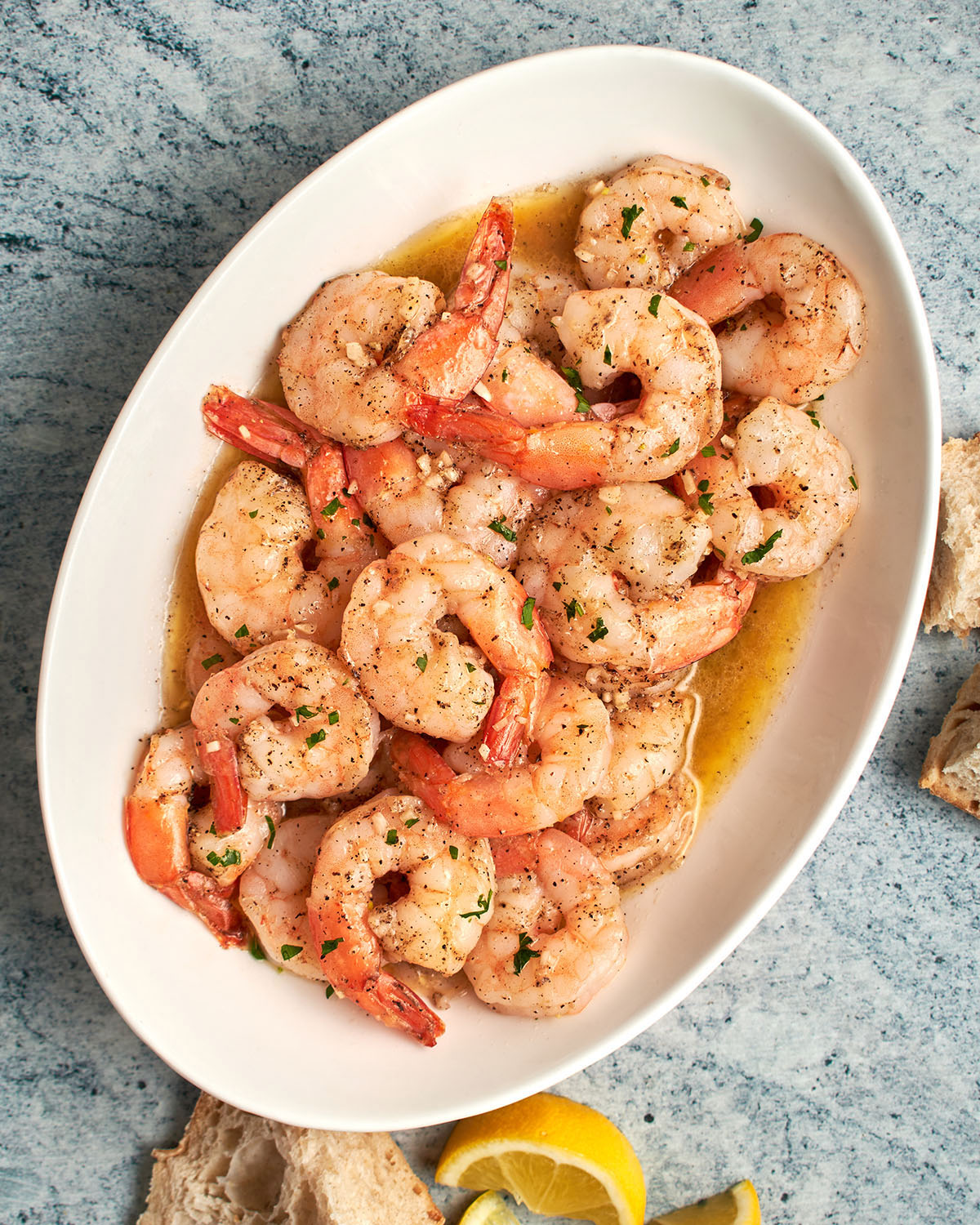This image is a color photograph, horizontally oriented, centered on a large white, oval bowl positioned at a diagonal angle with its bottom facing the lower left corner and its top toward the top right. The background features a white tabletop with blue dots. Inside the bowl, several light pink shrimp, with tails on and slightly darker towards the end, are arranged in a pool of light brownish-yellow liquid, likely butter. The sautéed shrimp are garnished with scattered green herbs and black pepper specks, adding a touch of freshness and color contrast. Resting in the bottom left of the bowl is a small piece of crusty bread and a lemon wedge with the rind side up. Additionally, more pieces of bread are visible underneath the bowl in the right middle portion of the image. The scene is captured from above, showcasing a delicately prepared dish of shrimp in a visually appealing manner.